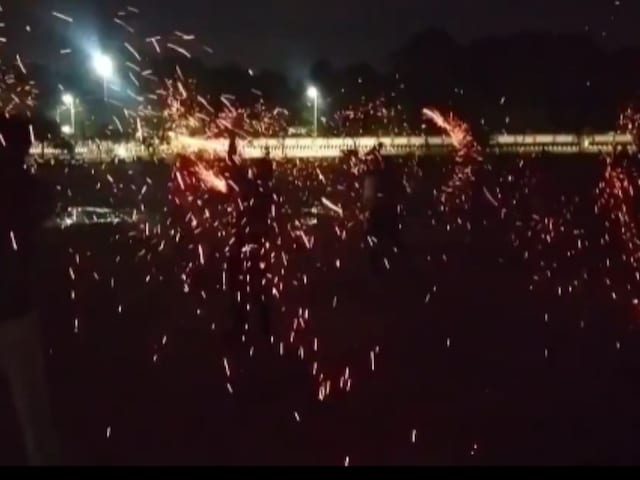This is an intriguing and somewhat surreal photograph of the Karthagai Deepam Festival in Tamil Nadu, taken during the night. The image captures a distant, narrow bridge or walkway with streetlights above it, casting a stark white illumination against the otherwise dark surroundings. Underneath the bridge, what initially appears to be fireworks or fire embers are actually people engaging in a traditional activity of the festival by waving Mavoli, which are branches with palms set aflame, creating circular, fiery displays. These bursts of light appear as yellow to reddish flashes, adding vibrant streaks to the photograph. The picture is extremely blurry, making it difficult to discern finer details, but a person can be seen in the background with one arm raised amidst the dark silhouettes of trees. The overall composition is vivid and mysterious, emphasizing the captivating but unclear scene depicted in the vibrant glow of the Mavoli and the distant, white streetlights above the bridge.